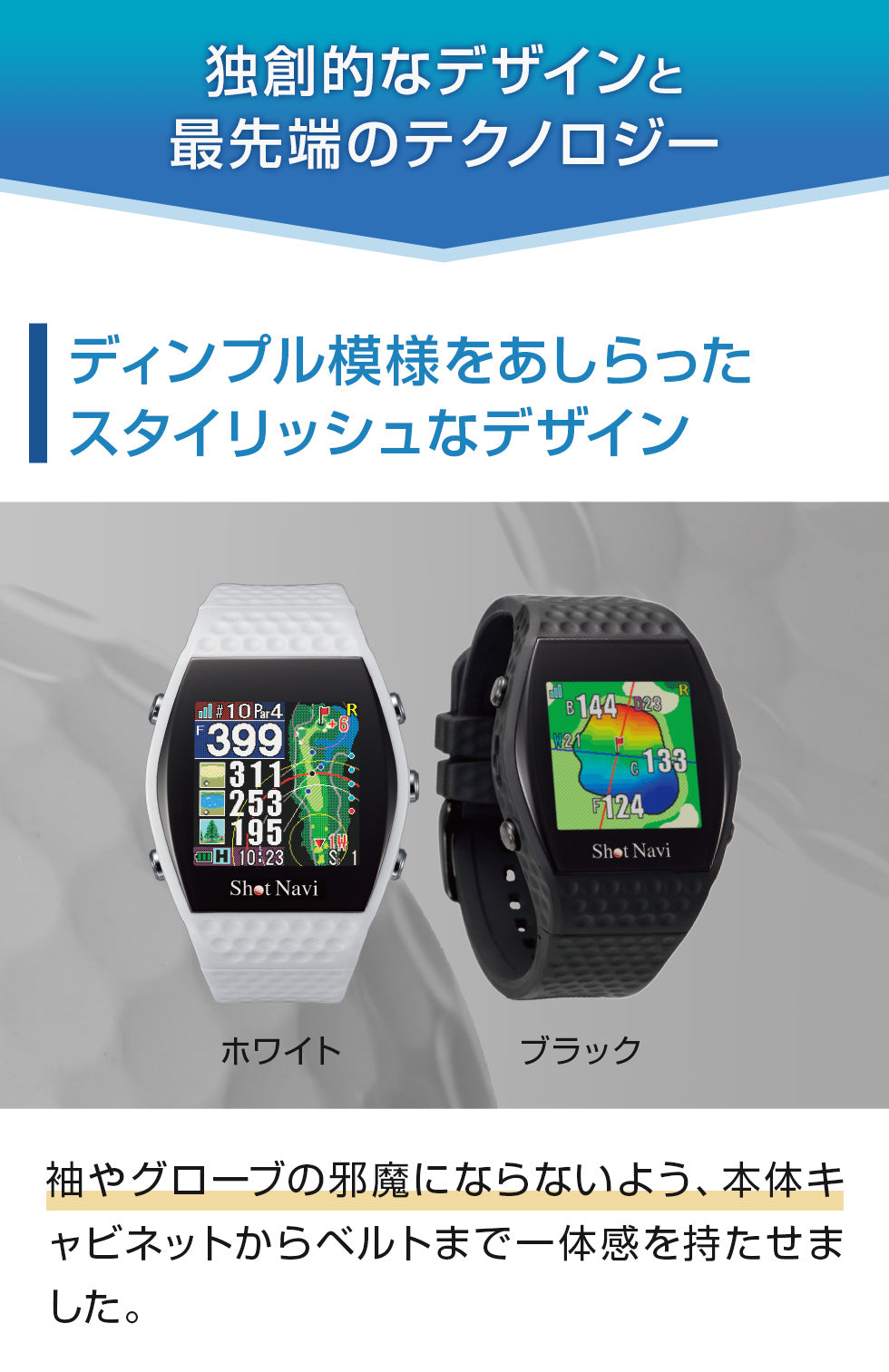This advertisement features two smartwatches side by side, one with a black band and the other with a white band, both sporting a unique, golf ball-like textured strap. The central image highlights their colorful, high-definition screens, displaying a golf-related app with details about the golf green, flag, distances, slopes, and scores. The brand name 'Shot Navi' is prominently displayed below the screens, indicating a specialized golf theme for these smartwatches. The background is a close-up image of a gray golf ball, reinforcing the golfing motif. The advertisement has text in Japanese above and below the watches, contributing to the overall aesthetic. The top section of the page is blue with white Chinese text, while the middle section is white with blue writing, transitioning to a white bottom section with smaller black text. The black smartwatch displays three numbers (144, 133, 124) with a red line and vibrant rainbow colors, and the white one shows four numbers (399, 311, 265, 195), emphasizing their advanced features.